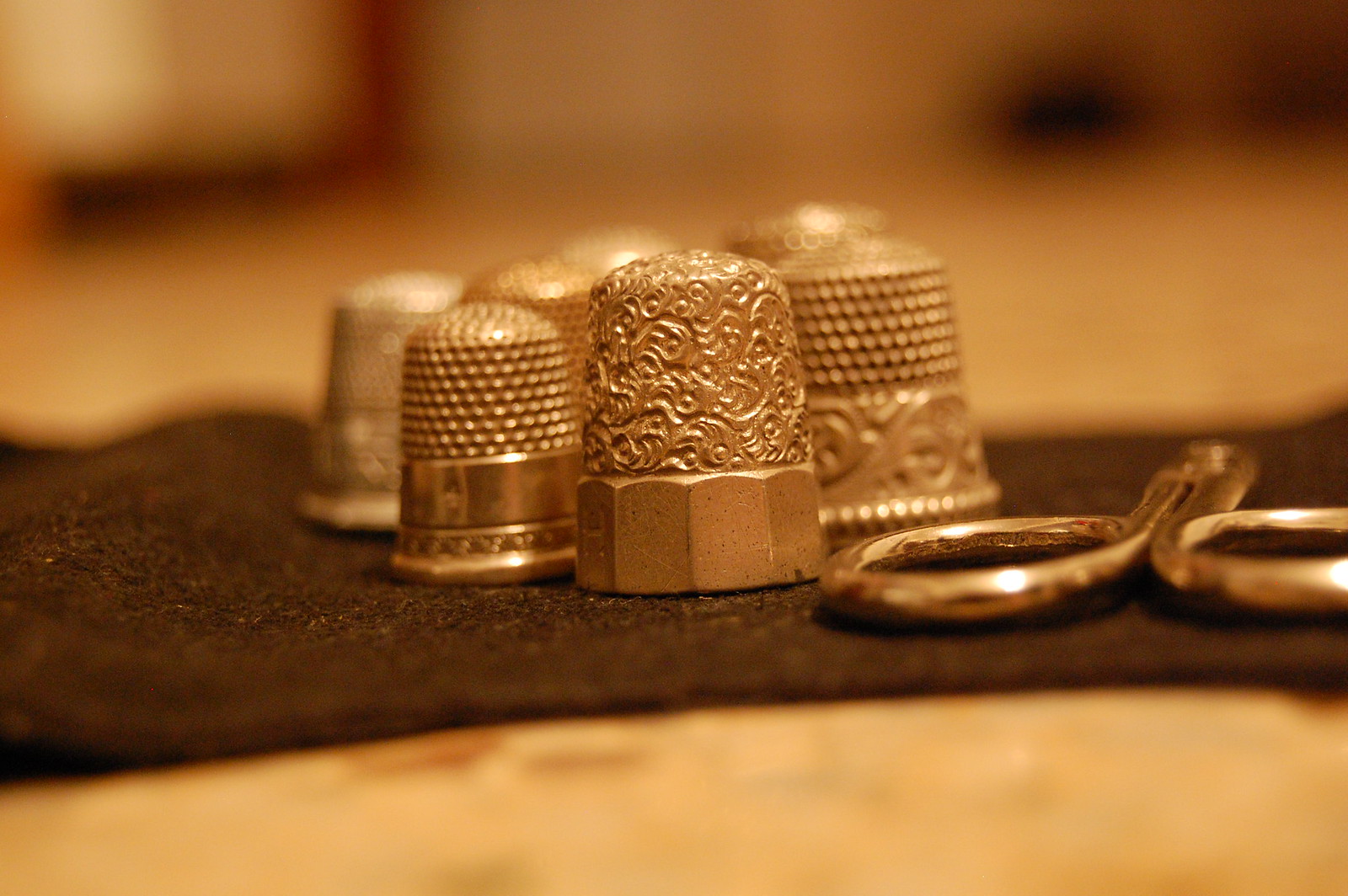The image depicts a set of intricately decorated sewing thimbles arranged standing upright on a black cloth that stretches horizontally across the center. The cloth is placed on a table, and we're looking at the scene from an eye-level perspective. The background is largely out of focus, presenting a blend of yellowish, pinkish, and whitish hues at the top, and similar colors along with some light brown shades towards the bottom.

In the center of the cloth, there are seven thimbles with varied designs and colors, primarily silver and gold. From left to right: 
- The first thimble at the back is small, silver, and out of focus.
- Slightly to the right and towards the front is a gold thimble.
- Behind the gold thimble is another gold one.
- To the left of this second gold thimble, barely visible, is the top of a silver thimble.
- Further to the left, another silver thimble's top is just visible.
- Front and center, there is a prominent thimble that resembles a metallic nut with squared-off sides at the bottom and detailed etchings on the top part.
- To the right, an ornate thimble features more elaborate carvings and a slightly ruffled design.

On the far right of the cloth, lying flat with the handles facing towards the camera, are a pair of silver scissors. The image captures the side and a bit of the top of the scissors, maintaining the eye-level view.